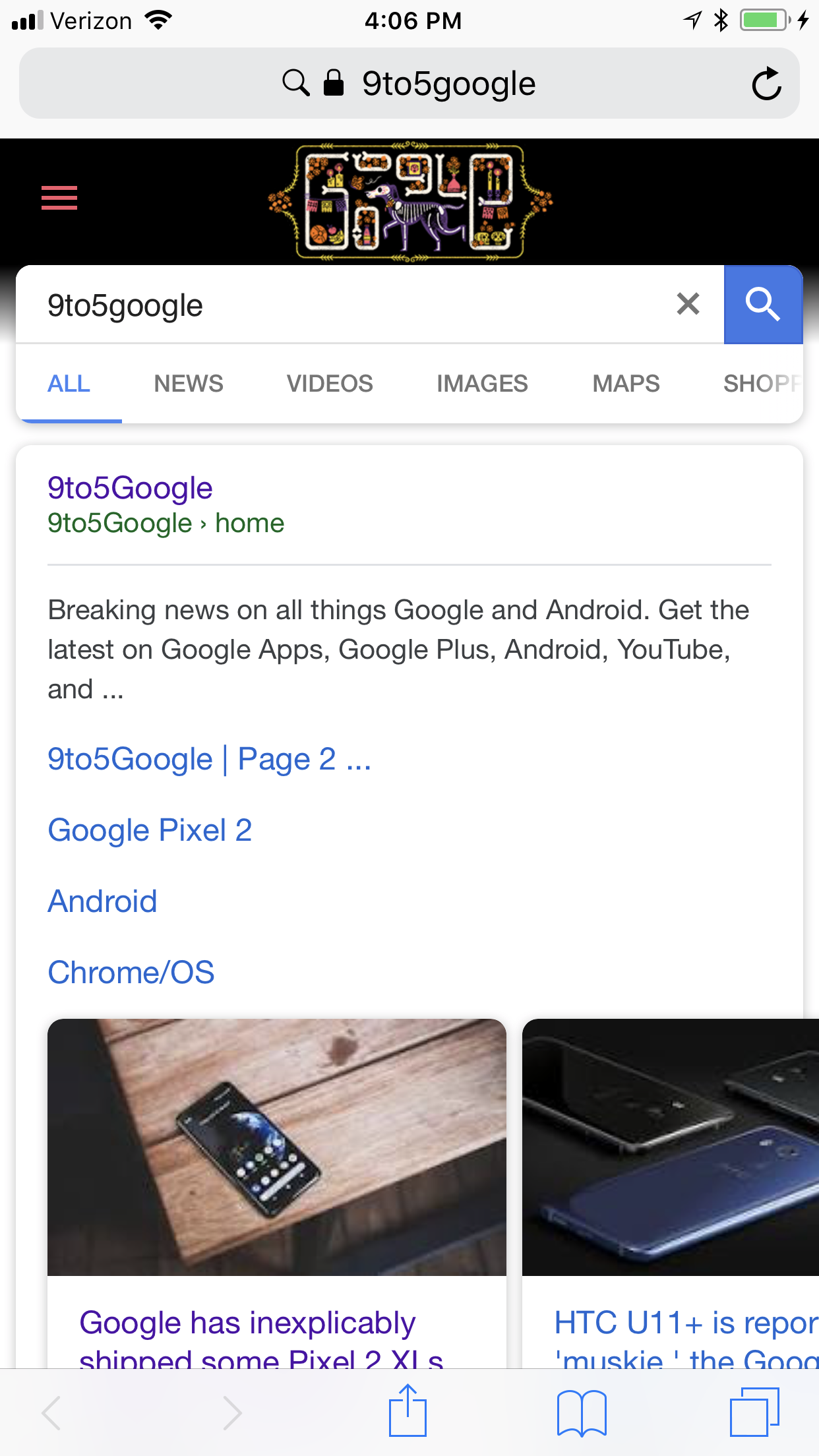A person is seen holding their phone, conducting a Google search for "9to5Google." The search results prominently display the official 9to5Google website, which is a platform known for breaking news related to Google and Android. The webpage offers the latest updates on Google Apps, Google+, Android, and other relevant topics. There's a section featuring additional embedded links, including articles about the Google Pixel 2, Android, and Chrome OS, and a mention that Google has unexpectedly shipped some Pixel 2 XL units, alongside information about the HTC U11.

The search results page retains the typical Google layout with a white background and blue hyperlinks. Users have the option to filter their search by categories such as news, videos, images, and maps. At the top of the page, there's a whimsical Google Doodle featuring a black background and the skeletal image of a dog, likely celebrating the Day of the Dead, adding a festive touch to the otherwise standard interface.